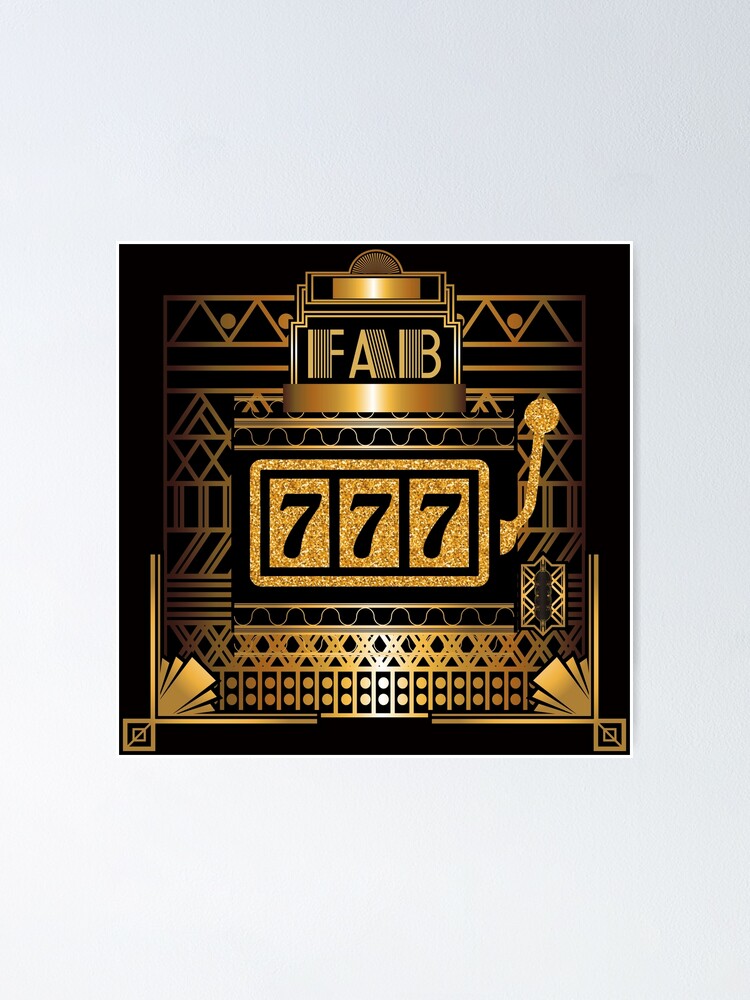This captivating image is a meticulously detailed illustration of a stylized, Las Vegas-style slot machine, rendered in a striking art deco style. Set against a rich black background, the slot machine is predominantly gold, creating a brilliant contrast. The centerpiece features the triumphant combination of three black sevens (777) framed in gold, suggesting a winning pull. To the right, a golden lever is depicted, emphasizing its slot machine identity. Geometric shapes, including triangles, wave motifs, and fan-like patterns, embellish the borders, enhancing the overall elegance. The top of the machine is adorned with the letters "FAB" in gleaming gold, adding to its opulent appearance. Additional details include a coin slot and illustrations suggesting the payout of coins. The piece, radiating with shiny gold elements against the dark backdrop, is presented with such clarity that it's hard to discern whether it's a photograph or a painting. The image, likely hanging on a gray or white wall, combines the allure of casino excitement with the timeless appeal of art deco aesthetics.